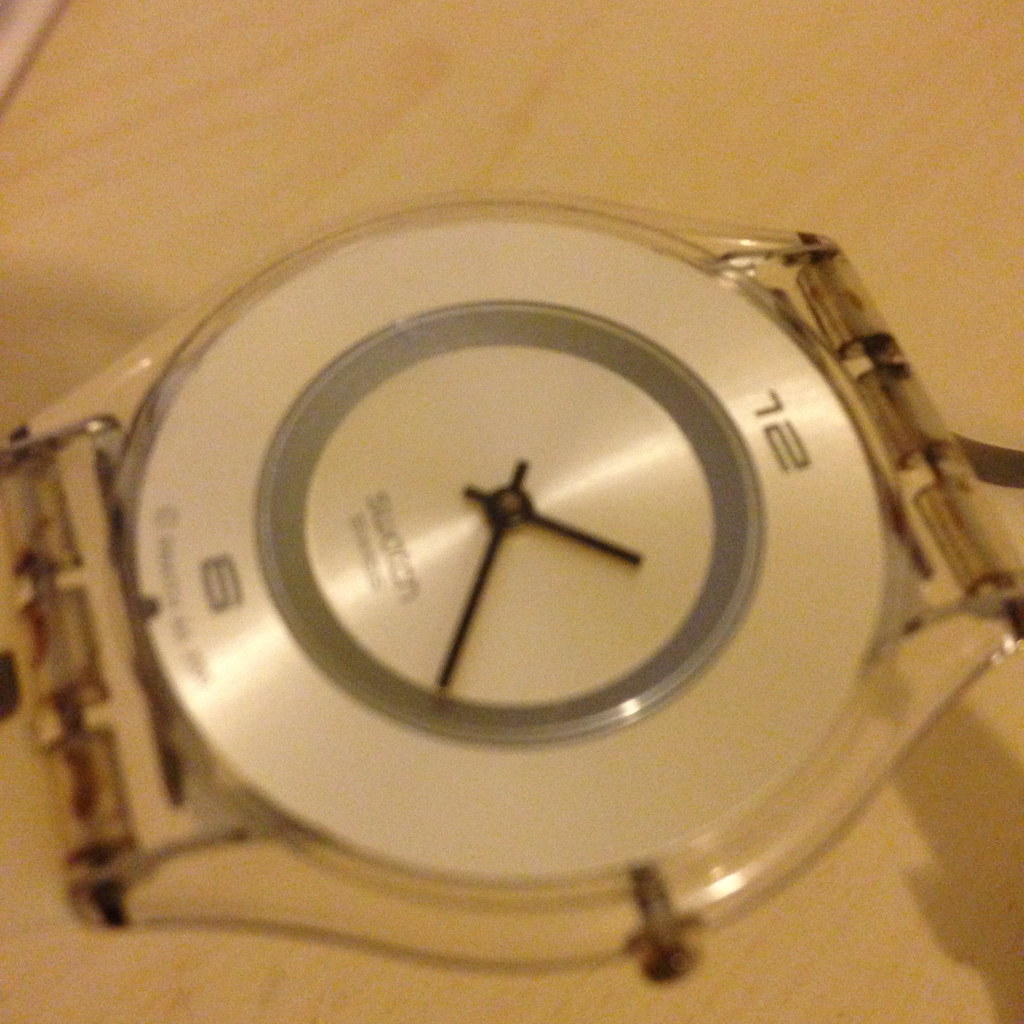The image features a Swatch watch with a round, clear plastic face that stands out against a light-colored wooden table with darker, textured tones, positioned at a diagonal angle. The face of the watch is a pearly white tone with only the numbers 12 and 6 above a small, central gray circle. While there are black hour and minute hands, they are thin and there is no second hand. Below the number 6, there is some gray text that is unreadable. The watch lacks straps and shows some signs of rust at the top and bottom, particularly around the wind-up knob, indicating slight wear. The dial appears to point to around 2:25.